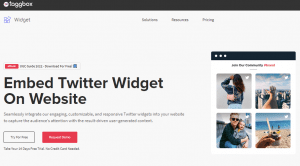This is a screenshot of a webpage from Tagbox. The page is titled "Embed Twitter Widget on Website," displayed prominently in large black text at the top. In the top left corner, the word "Widget" is clearly visible. Below the main title is smaller text that is unfortunately too blurry to read. 

Beneath the smaller text are two buttons: the one on the left likely says "Try It Now," while the one on the right is a prominent pink box with white lettering, which also includes another line of text beneath it that is not legible.

On the right side of the screenshot, there is a browser window displaying four photographs. The first photograph shows a woman facing a wall; she is wearing a printed blouse and carrying a small purse over her shoulder. The second photograph captures a view from a skyscraper. The third image depicts a father and daughter posing for a picture on a road. The fourth and final photograph features a beach background with a close-up of a dessert, possibly a gelatin or ice cream, held by a person.